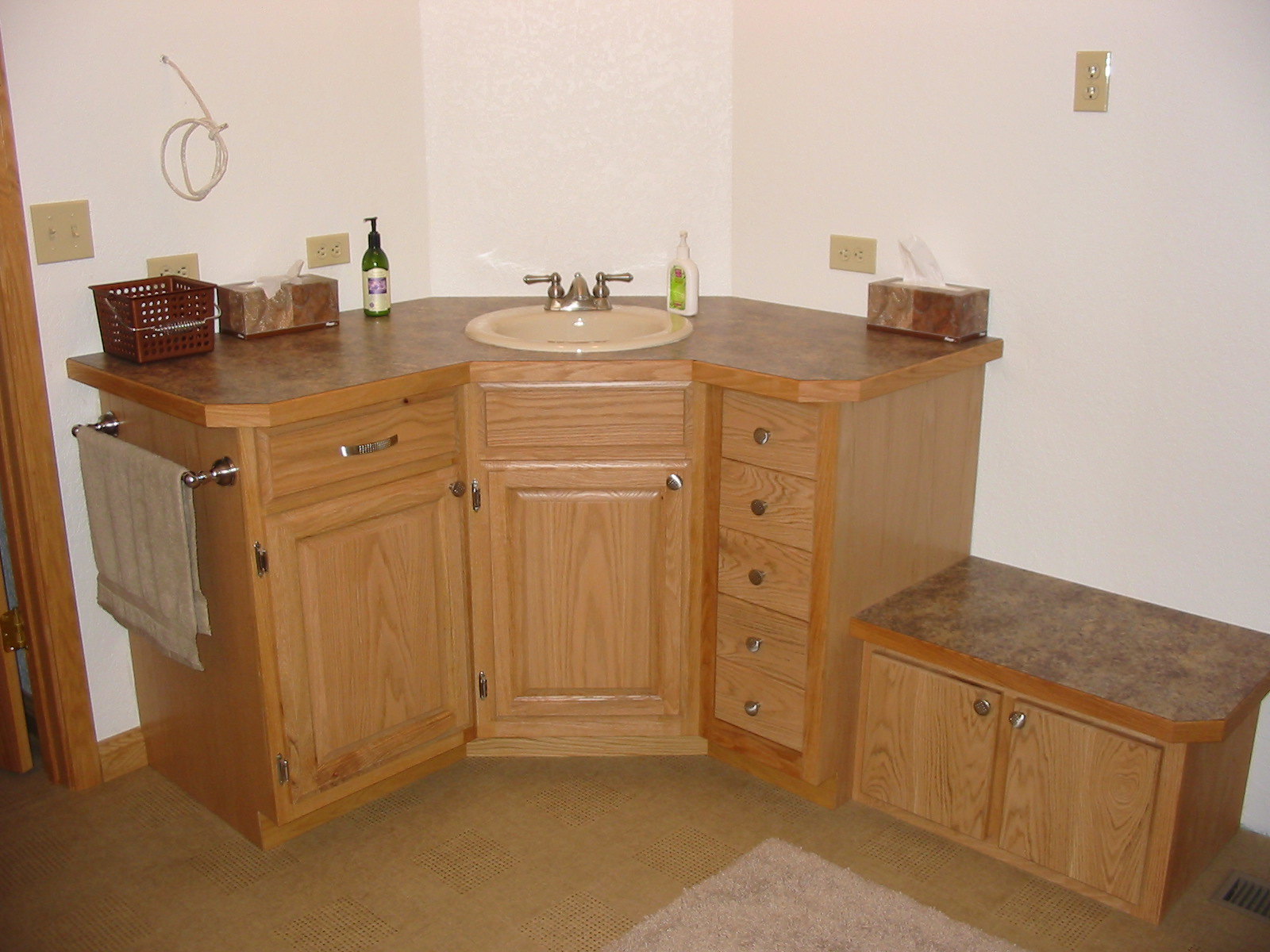This photograph showcases a bathroom styled from the 1970s or 80s, situated in a corner with an angled design. The cabinetry is made of oak and features vintage details. There are two cabinet doors and six drawers in total. On the right side are five narrow, vertical drawers, while the left side has one wider drawer positioned above a cabinet door. Beneath the sink, which is centrally located on the angled corner, there's another cabinet door. The sink itself is a light brown or tan color and is fitted with an 80s-style brass faucet.

On the countertop, which appears to be adorned with a fake burl Formica surface trimmed with oak, there are two boxes of Kleenex placed on either side. To the right of the countertop is a much lower cabinet with two front doors, topped with the same Formica surface, and sitting at the height of a chair.

The background features white walls, with a door to the left framed in oak trim. Adjacent to the door, there are two light switches and a coiled wire, possibly for an old phone. Additionally, there are two electrical outlets: one on the left side and a double outlet on the right side.